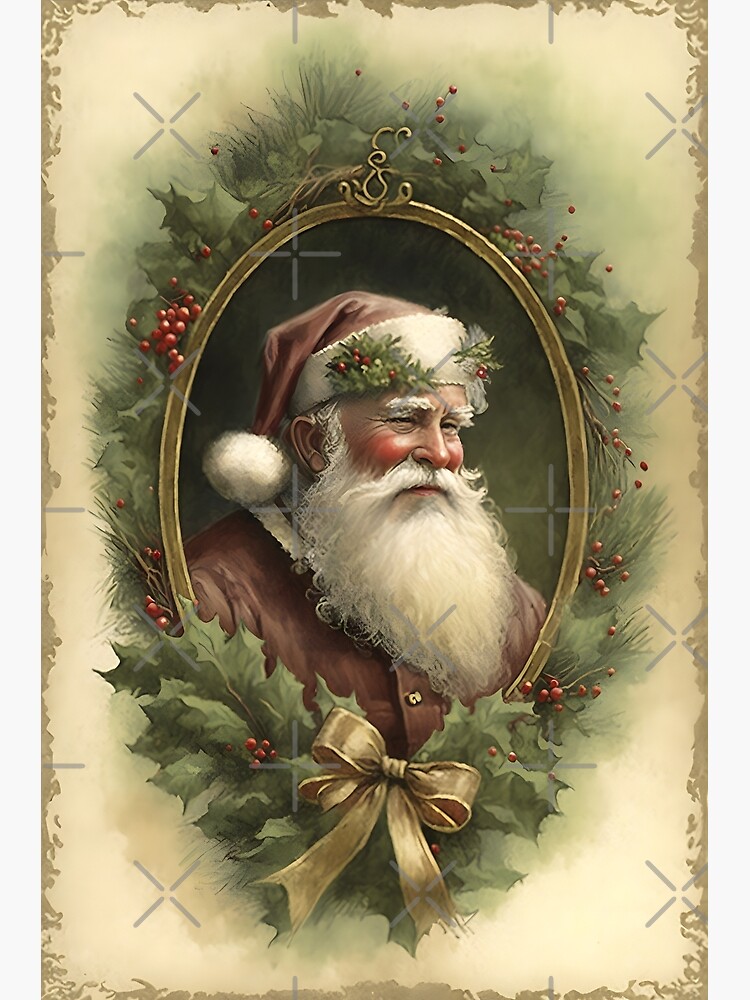This artwork portrays a vibrant and detailed portrait of Santa Claus centered within an embellished gold oval frame. The frame is adorned with an intricate wreath of pine leaves, oak-like leaves, and prickly Christmas bushes featuring red berries. A gold ribbon ties the wreath together at the bottom, providing a festive touch. Santa Claus is depicted wearing his iconic red hat with a white fur trim and a white ball on the end, as well as his signature red coat with gold buttons. His rosy cheeks, bushy white beard, and thick white eyebrows lend him a jovial appearance as he smiles warmly. The background of the image is predominantly a creamy white, contributing to the bright and clear presentation of the scene. No text or numbers are present in the image, ensuring the focus remains on the cheerful depiction of Santa Claus within the festive wreath.